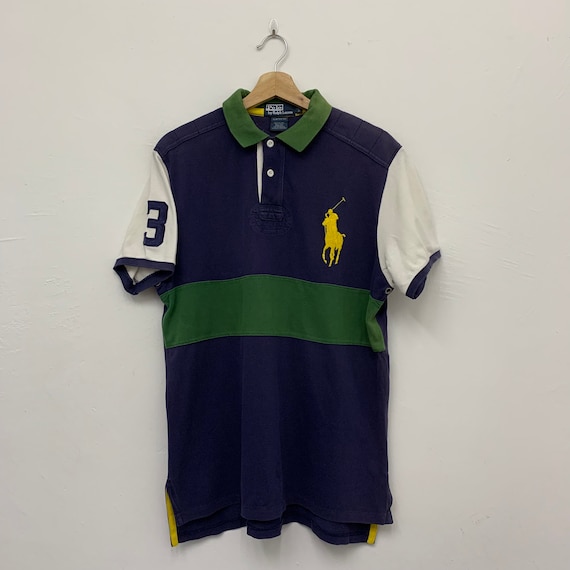The image depicts a well-worn Ralph Lauren polo shirt hanging on a wooden hanger with a metal hook, which is attached to another hook emerging from a white wall. The shirt features a green collar with two buttoned buttons and short white sleeves adorned with dark blue trim. Its design is divided into three sections: the top half is blue, the middle features a prominent green stripe, and the bottom half returns to blue. Yellow slits are visible on each side of the shirt. On the front left chest, there is a yellow illustration of a polo player on a horse. A large number three is emblazoned on the right sleeve. The image shows some shadowing against the wall, suggesting it may be intended for resale on a classifieds ad or social media platform.